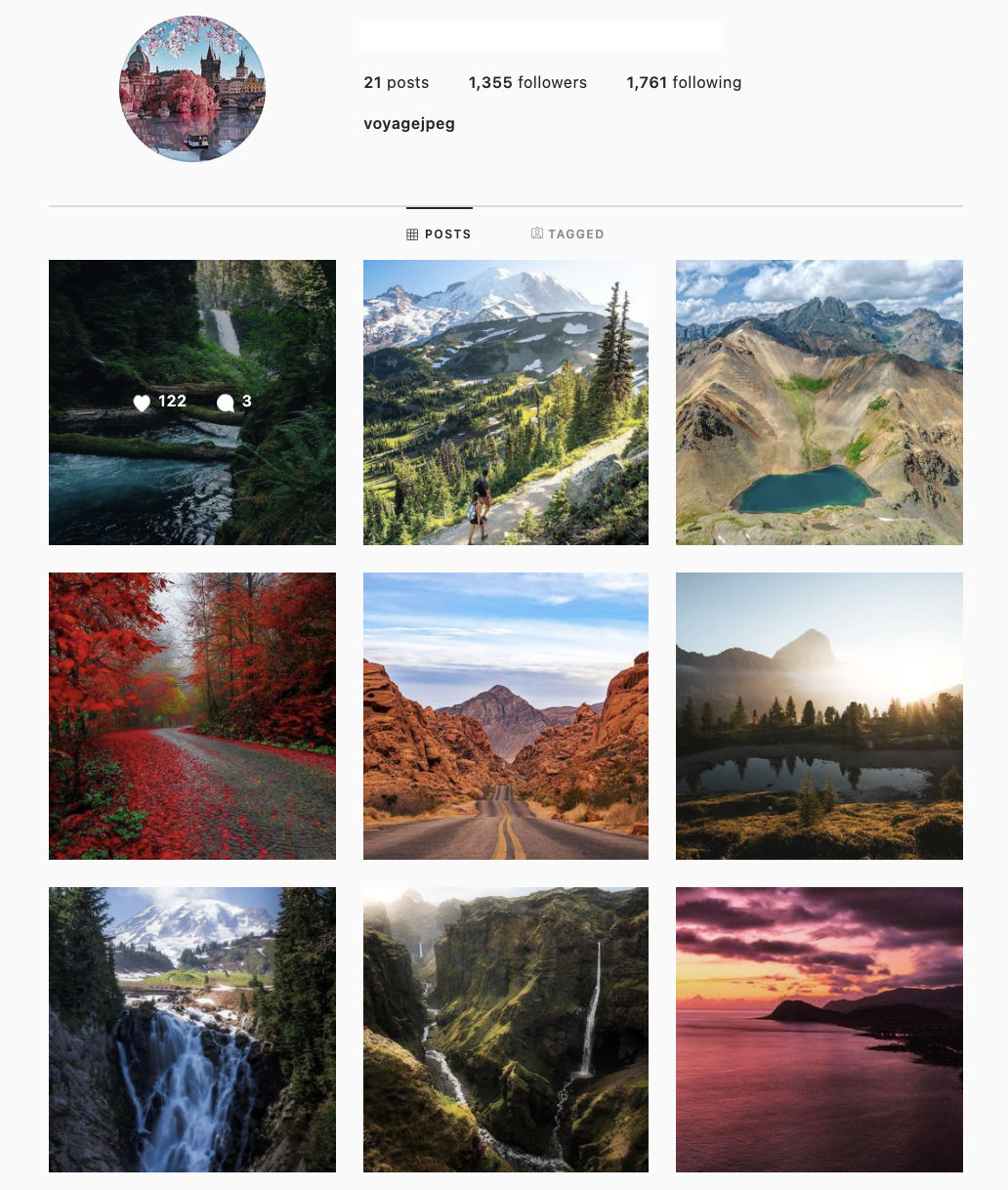The image showcases a social media profile dedicated to scenic photography. At the very top, there's a profile icon featuring a distant body of water, framed by pink leaves and a blue sky. To the right of the profile icon, text indicates "21 posts," "1,355 followers," and "1,761 following." Directly below, the username "voyage.jpeg" is displayed. 

The profile features two tabs, "Posts" and "Tagged," with "Posts" currently selected, displaying a grid of nine images. 

Starting from the top left:
1. An image of a serene body of water surrounded by dark leaves, with a heart icon showing 122 likes and three comments.
2. A video of a person standing at the edge of a mountain, capturing a breathtaking view.
3. A photograph of mountainous terrain.

In the middle row:
4. A picturesque road flanked by vibrant red leaves, emblematic of the fall season.
5. Another road framed by rugged mountainous edges on both sides.
6. A tranquil pond with trees and sunlight in the background.

On the bottom row:
7. A stunning waterfall with mountains looming in the distance.
8. Two rivers winding through a mountainous landscape.
9. A captivating image of a purple sunset casting its hues over a body of water.

Each image exudes an essence of natural beauty, encapsulating various picturesque landscapes and moments.